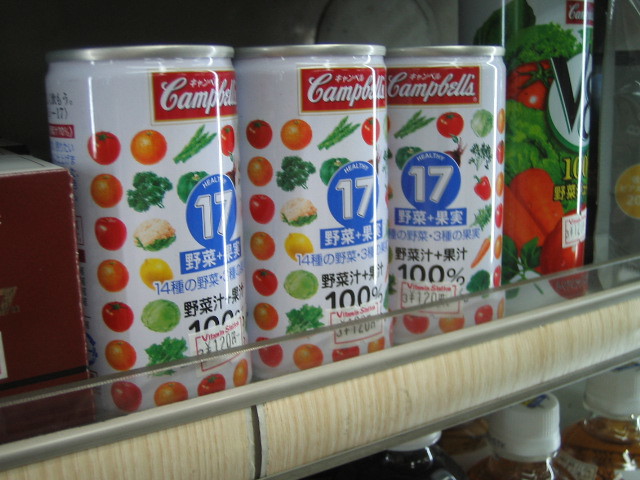This image captures an angled close-up view of a store shelf stocked with various cans and bottles. Prominently displayed are three white cans of Campbell's soup, featuring colorful imagery of fruits and vegetables. The cans bear the classic Campbell's logo, with a red square housing white lettering at the top. In the center of each can, there's a distinctive blue circle containing the numeral 17 and Asian characters, suggesting these might be foreign products. Below the blue circle, a blue rectangle is present. To the right of the Campbell's cans is a notably larger V8 can, which displays partial imagery of carrots, tomatoes, and lettuce along with the recognizable V8 logo. Beneath the shelf, partially visible on the bottom right, are what appear to be two goldish bottles with white caps, possibly apple juice. An additional element in the bottom left corner is a gray border of the shelf structure, angled upward to the right, with a thin plastic strip running across it. To the far left, a small red and white square box is partially in view. The setting appears to be a convenience store or refrigerated cooler, indicated by the absence of visible price tags on the items.